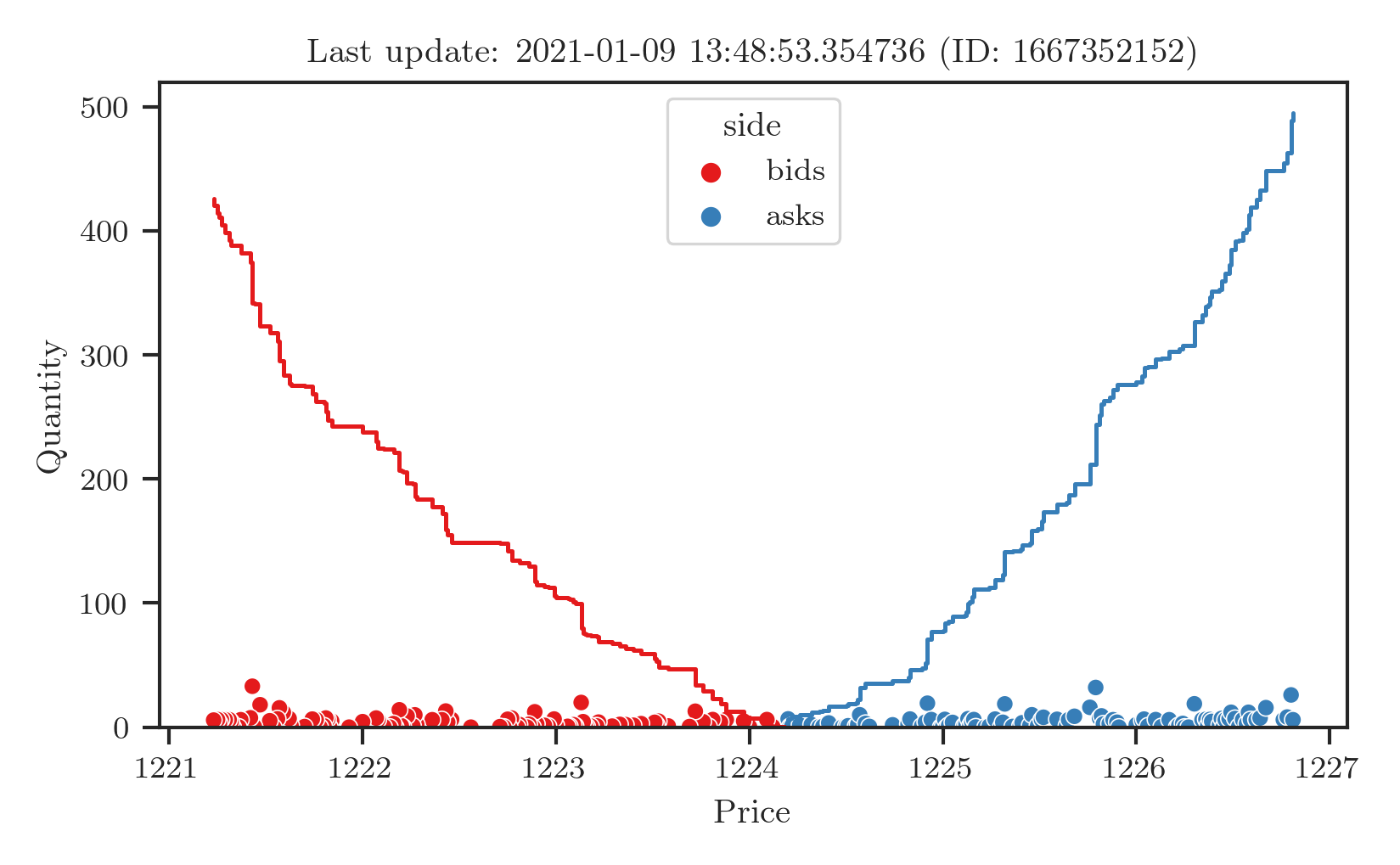The image depicts a detailed price chart within a thin black-bordered box, last updated on 2020-01-09 at 13:48:53.354736, with an ID of 1667352152. The horizontal axis at the bottom of the chart is labeled "Price" and ranges from 1221 to 1227. The vertical axis on the left side is labeled "Quantity," with values incrementing by 100 from 0 to 500. 

Within the graph, there is a key enclosed in a gray box labeled "Side." This key includes a red dot for "Bid" and a blue dot for "Ask." The chart shows a series of red dots (bids) declining from a quantity of 400 at a price of 1221 to 0 at 1224, forming a downward slope on the left side of the graph. Conversely, blue dots (asks) increase from a quantity of 0 at 1224 to nearly 500 at 1227, forming an upward slope on the right side, characterized by a jiggly, zigzagging pattern.